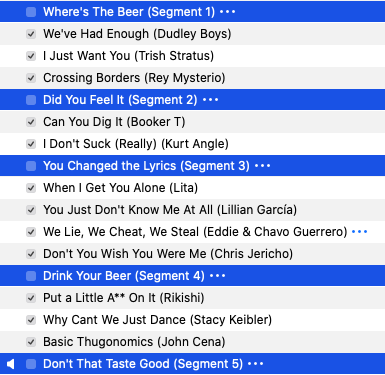This image is an older screenshot, possibly taken from a mobile device, an iPad, or a cropped desktop view featuring an interface that resembles iTunes or a similar media application. The interface displays a list of items, with alternating row colors reminiscent of older iTunes versions: one row is light gray, followed by white, and so on. However, in this screenshot, the rows are highlighted in blue, indicating selection. 

The list comprises various segments:

1. "Where's the Beer? Segment 1"
2. "Did You Feel It? Segment 2"
3. "You Changed the Lyrics? Segment 3"
4. "Drink Your Beer? Segment 4"
5. "Don't That Taste Good? Segment 5"

On the left-hand side, there are options to select each segment, suggesting that all sections are currently selected, which is why they are highlighted in blue. At the very bottom, next to "Don't That Taste Good? Segment 5," an audio icon is visible, likely indicating playback or audio options for that segment.